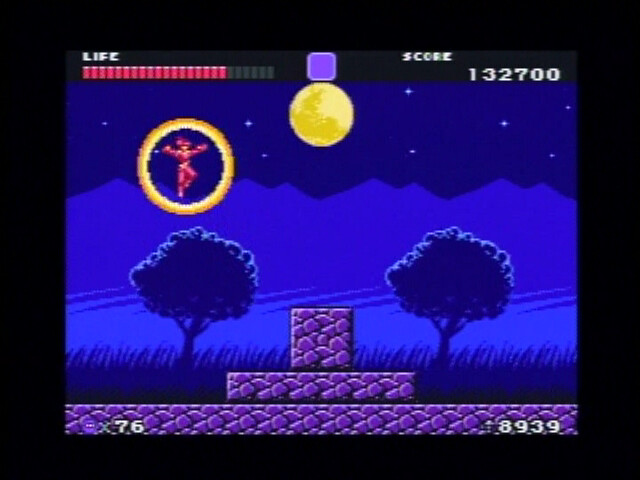This image depicts a classic early era video game, likely from a Nintendo console, framed by a black border. At the top of the screen, a red life bar is displayed, just below which, in the top right corner, a white score counter reads "132,700." The scene portrays a nighttime setting under a sky adorned with a bright yellow moon positioned in the top center, accompanied by scattered clouds and twinkling stars. Dominating the midsection of the screen is a red character, seemingly flying within a yellow circular border. This character is flanked by two identical trees—one on the left and one on the right. Additionally, there are several purple blocks scattered across the scene, adding to the game's environmental obstacles. The lower left corner of the screen features the number "76," while the lower right corner displays the numbers "89" and "39."